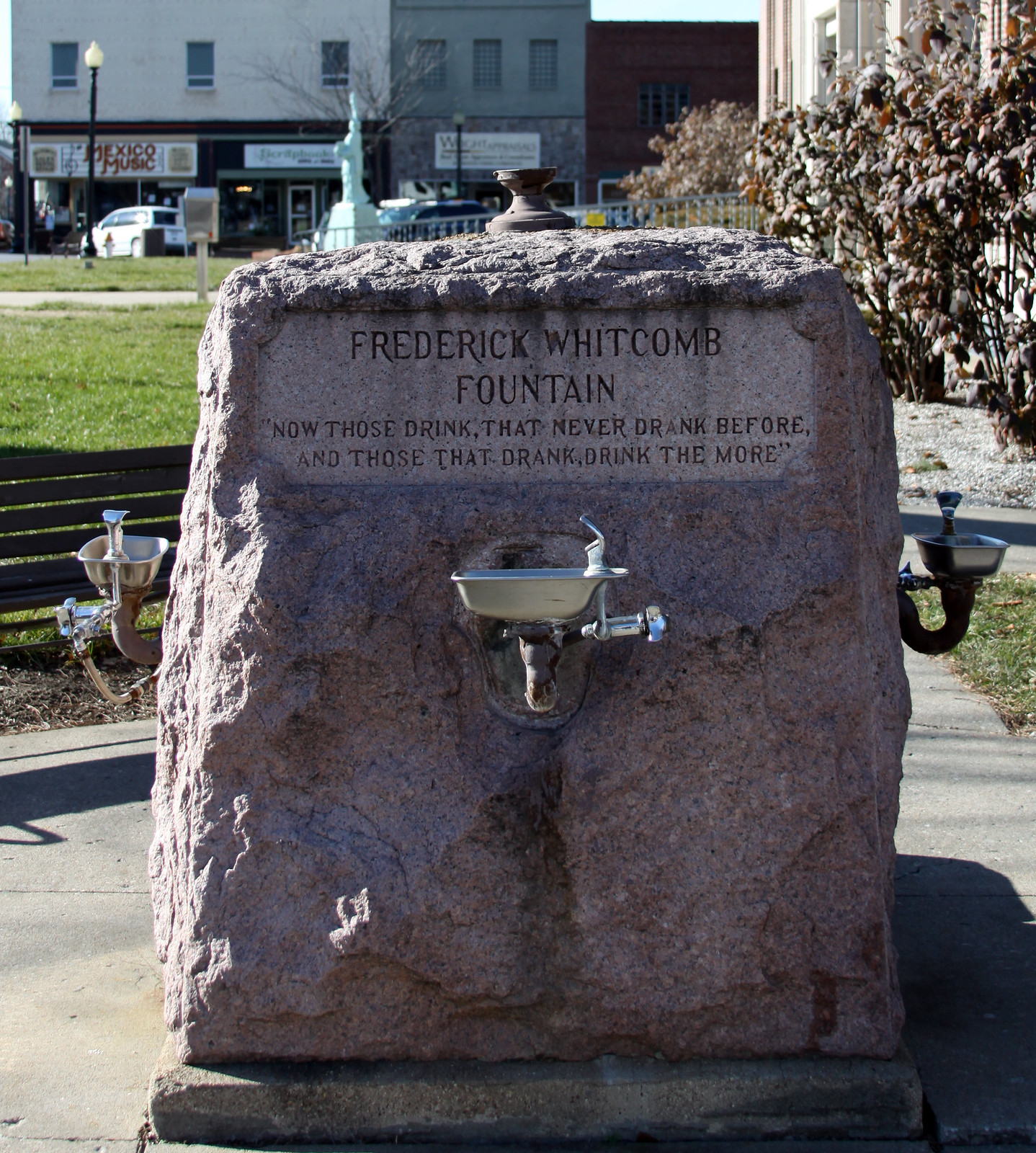This photograph showcases the Frederick Whitcomb Fountain, centrally positioned in a city park. The fountain is a large, gray stone structure featuring three stainless steel water spigots on the left, center, and right sides for drinking. The stone is engraved with the text: "Frederick Whitcomb Fountain. Now those drink that never drank before, and those that drank, drank the more."

The background reveals a bustling cityscape with various buildings, including a music shop named "Mexico Music," identifiable by its prominent signage. In front of the shop, a white station wagon is parked, adding to the urban atmosphere. Surrounding the fountain, green grass and a neatly paved sidewalk can be seen, along with streetlamp posts and park benches. To the right of the stone, there's a tree with brown leaves, indicating a touch of nature in the urban setting. The entire scene is framed by additional city buildings in shades of white, gray, and brown, presenting a vibrant and detailed blend of natural and urban elements.